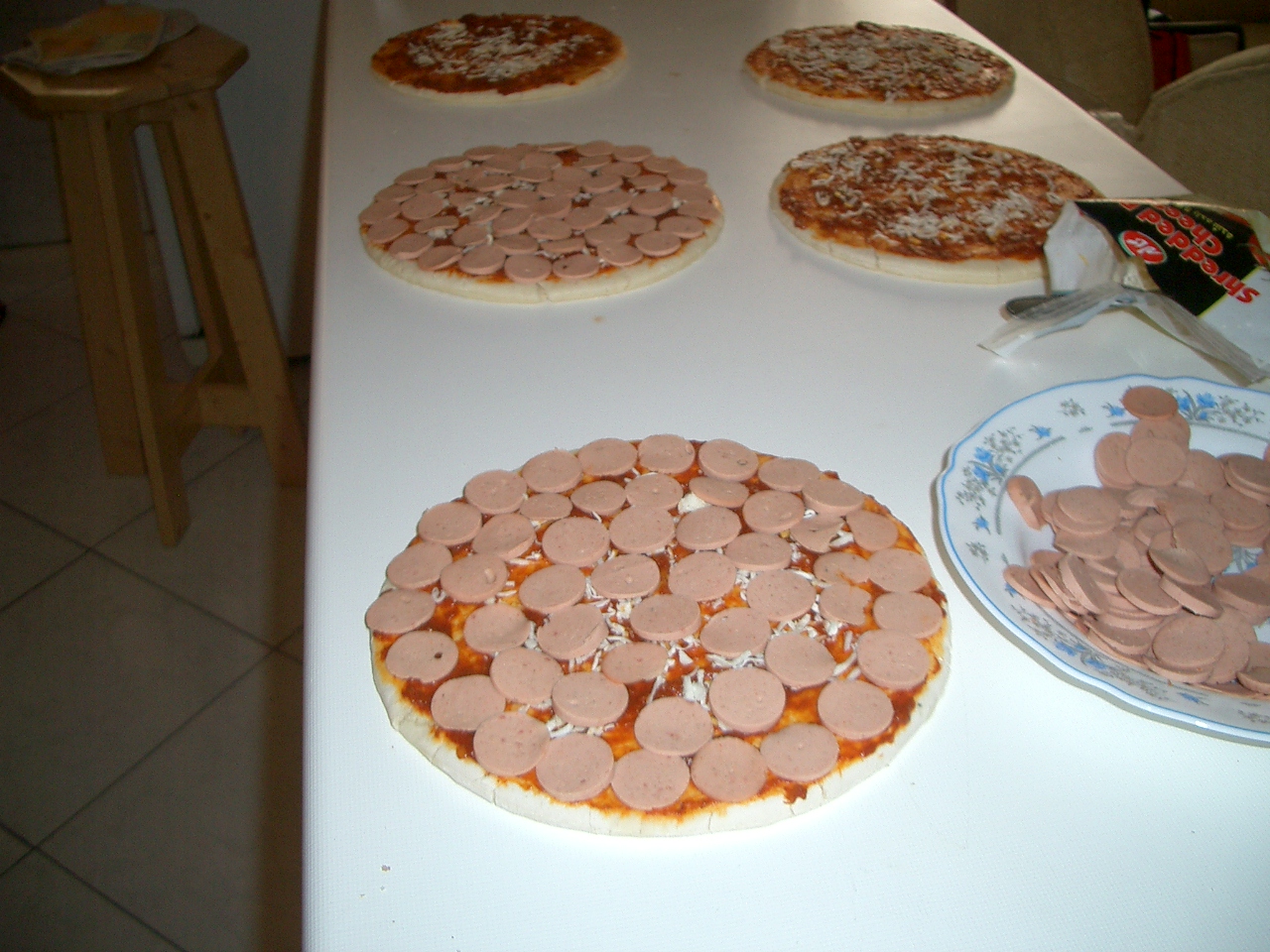The photograph showcases a long, white table set on a tiled floor with a high wooden stool in the upper left corner. The table is laden with five large pizzas, all featuring tomato sauce and cheese. Three of the pizzas, located towards the back, are simply adorned with cheese, while the two pizzas at the front are topped with slices of bologna, resembling ham or hot dog slices. Adjacent to the front pizzas is a white plate with a blue and grey floral rim, piled high with additional bologna slices. In the upper right corner of the table sits a partially open plastic bag incorporating red, black, and white colors, though its contents are unclear. The scene extends to a lightly visible chair edge in the top right, alongside additional wooden stools surrounding the table. The overall setting features a contrast of dark brown tiled floor against the light and structured tabletop arrangement.